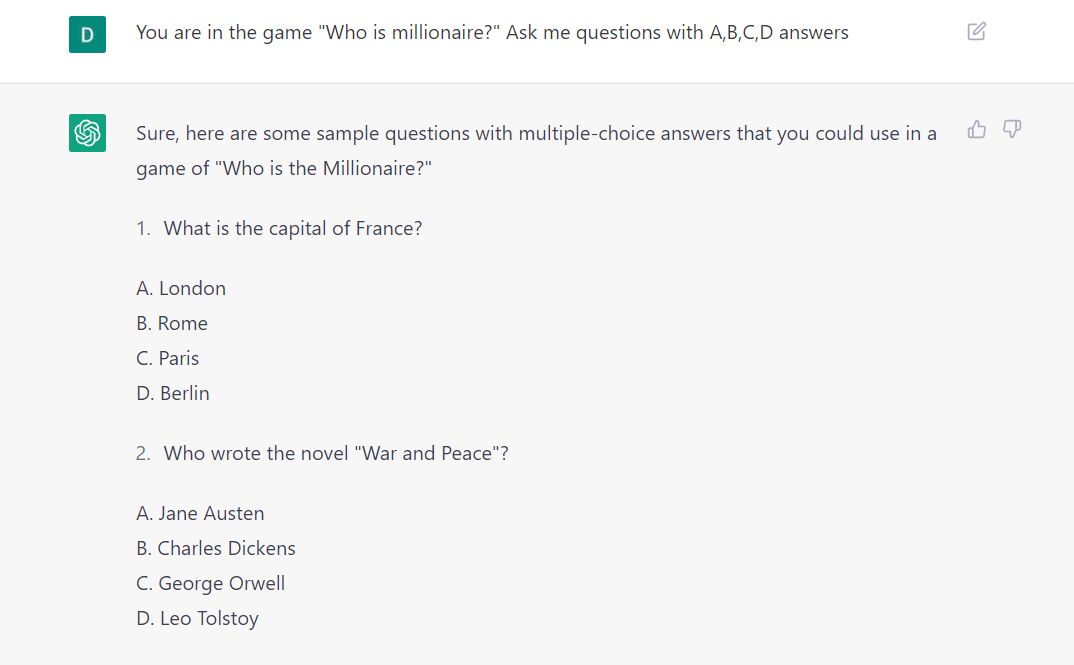The image features a white bar spanning across the top with black text that reads, "You are in the game. Who is a Millionaire? Ask me questions with A, B, C, D answers." To the right of this text, there's a small grey icon—a square with a pencil emerging from its upper right corner. To the left of this icon, there's a green square with a white "D" centered inside it.

Below this banner, the background shifts to a light grey hue. The section contains two questions. Preceding these questions, a heading states, "Sure, here are some questions with multiple choice answers that you could use in a game of Who is the Millionaire." The first question displayed is, "What is the capital of France?" accompanied by four multiple-choice options: A) London, B) Rome, C) Paris, and D) Berlin.